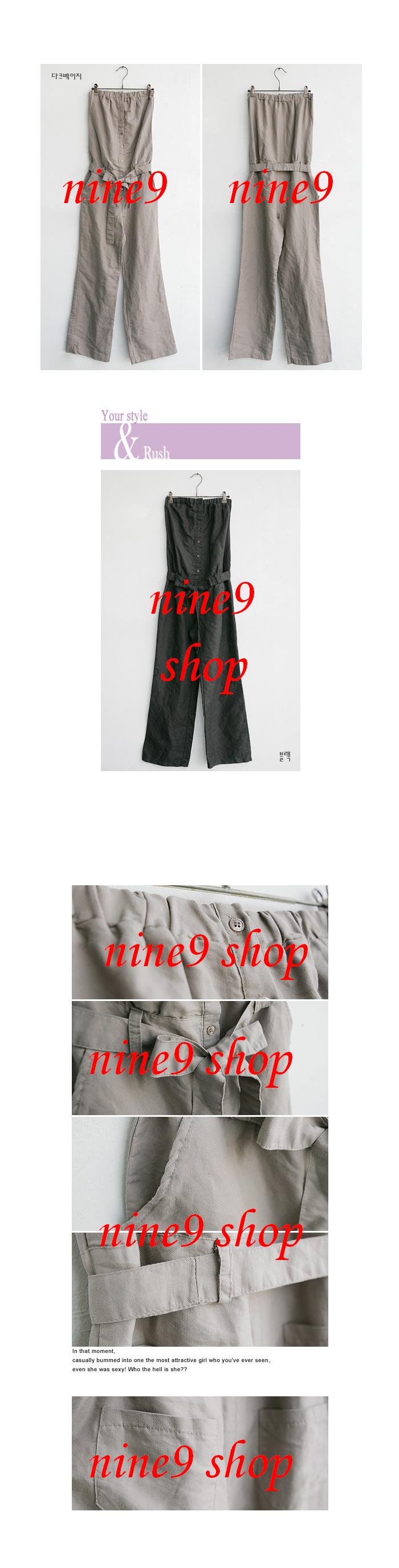The image is a series of six color photographs of women’s clothing, likely intended for an online or print catalog. The garments, which appear to be jumpsuits or dungarees, are in shades of gray and black. Each photograph features the text "NINE9 SHOP" in red italics, with "NINE" written out, followed by the number "9" and then the word "SHOP." The photos are organized in a collage, with some pictures showing close-ups that highlight specific garment details such as belts, waistlines, and the tops of the jumpsuits. Each item is displayed as if hanging on a hanger, but the hangers are laid flat on a table for the photographs. There is some very small, unreadable text on one of the images.